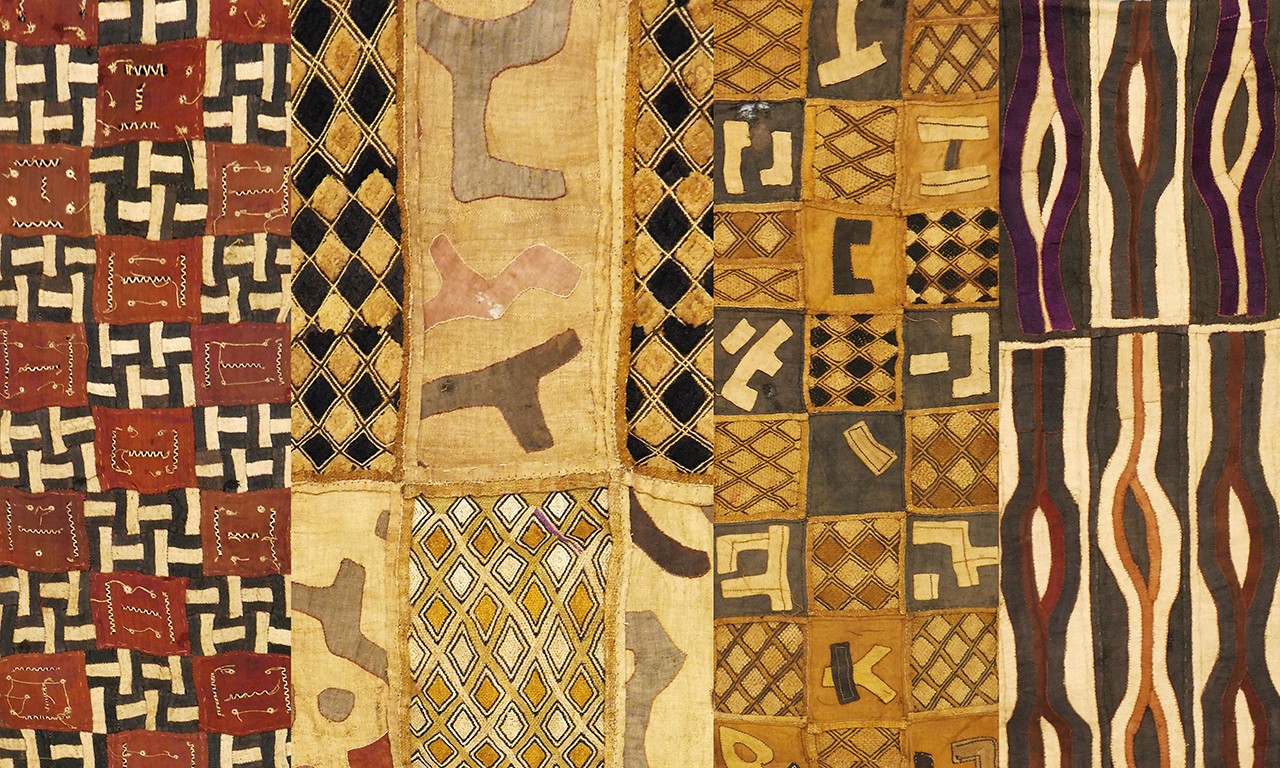This image displays an intricately designed, abstract artwork resembling a handmade quilt or blanket, featuring a multitude of vibrant patterns and symmetrical shapes collaged together. The composition includes a variety of colorful sections: 

On the left side, there are red squares with thin white patterns interspersed with black squares containing white sideways Ts. Adjacent to this pattern is a design of alternating black and gold diamonds, both horizontal and vertical. Beside that is a beige background adorned with shapes reminiscent of whale tails, presented in light blue, pink, and brown. 

To the right, another section showcases a series of squares. Some squares exhibit blackish-gray swirls with white dots inside, while others highlight gold and black diamonds, similar in pattern but varying in color. A prominent row of black diamonds interconnected by two thin yellow lines sits next to rows featuring yellow and white diamonds. The far right section contains squares with diverse backgrounds—white, black, or brown—decorated with ornate, belt buckle-like designs in white and yellow or black and red.

Overall, the piece is a rich tapestry of colors including red, brown, black, and orange, with an impressive array of shapes such as rectangles and diamonds, echoing the intricate craftsmanship typical of an African-designed quilt.